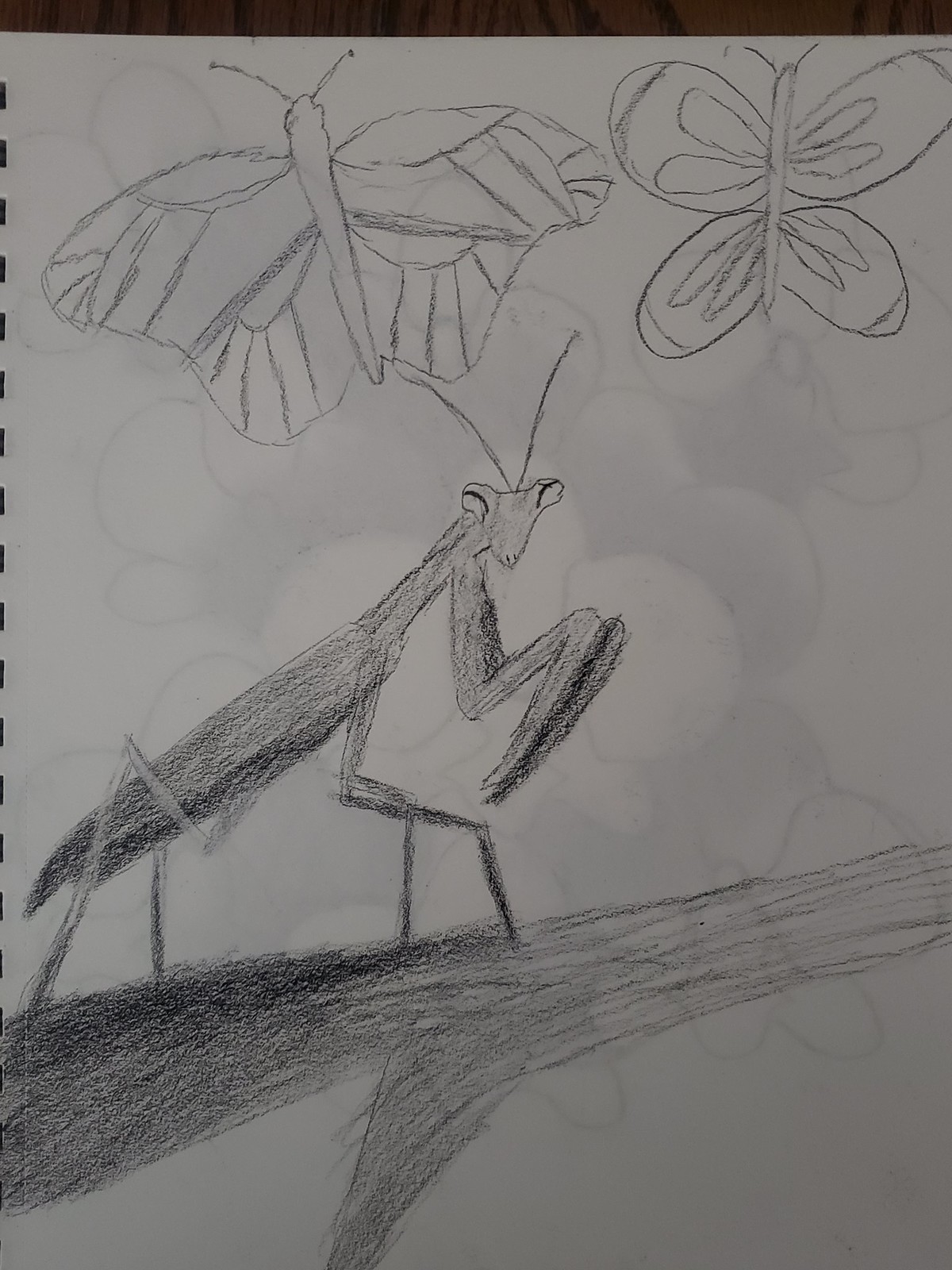This intricate pencil sketch, rendered on a sheet of spiral-bound sketchbook paper, features a detailed depiction of a praying mantis poised on a branching limb. The limb slopes from left to right and includes an extra offshoot extending towards the bottom center, meticulously shaded to enhance its realistic texture. The mantis, oriented sideways on the branch, gazes directly at the viewer with an almost lifelike intensity. The artist’s skillful shading captures the mantis’ intricate anatomy, including its two elongated antennae and precisely drawn legs—particularly its notable front limbs, resembling a bird’s beak.

Above the mantis, two butterflies, drawn with a simpler, less shaded technique, appear to be fluttering in the air. The butterfly on the left has one continuous wing outline and a worm-like body with thin antennae, while its counterpart on the right features a more traditional four-wing structure with oblong circles drawn on each wing. The subtle shadows and visible binding of the sketchbook add depth to the image, while faint impressions of another drawing are noticeable through the paper, suggesting an overlay from the reverse side.